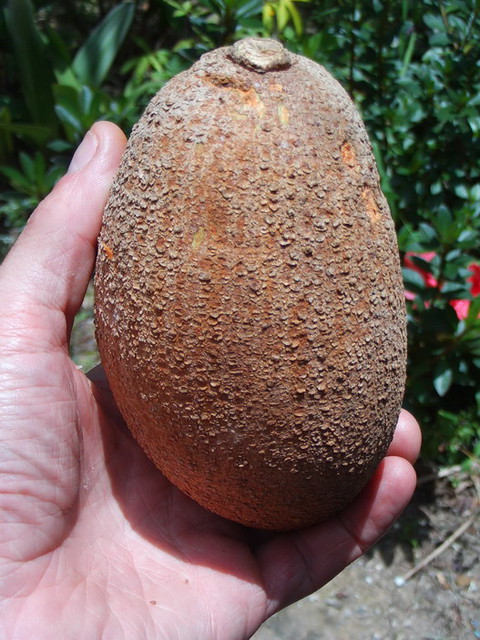The image captures a close-up of a Caucasian man's left hand holding an oblong, brown, scaly fruit, likely a mamey apple. The rough-skinned fruit, about the size of the man's palm, has horizontal lines and scars, and a stub at the top, indicating it was freshly picked. The man grips the fruit with his thumb on the left and fingers wrapped around the right side. The background reveals a lush green forest with leafy plants, some adorned with orange flowers, suggesting a natural and possibly tropical setting. The ground beneath is a mix of brown and grayish dirt or gravel, further enhancing the impression of an outdoor, garden, or jungle environment.